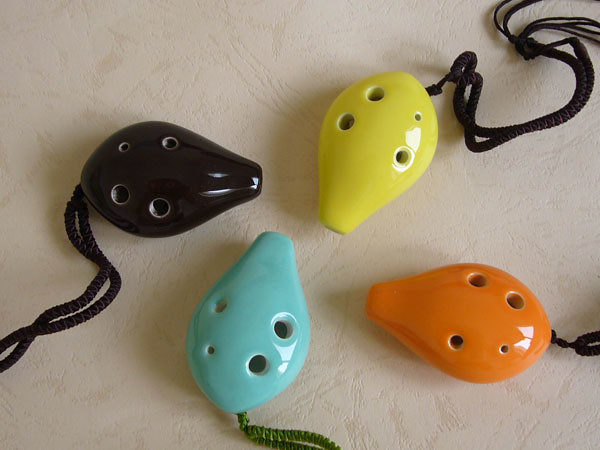This is an overhead colored photograph showcasing four ceramic objects arranged symmetrically on a white textured surface, which resembles a lightly embossed patterned paper. Each ceramic piece is identical in shape, reminiscent of hedgehogs or neti pots, with their 'faces' pointing inward toward a central point and their rounded bodies radiating outwards. Each object features three uniform-sized holes and a smaller hole on top. The ceramics are connected to short braided lanyards, suggesting they can be worn around the wrist or neck. The arrangement follows a clockwise color sequence: a glossy black ceramic at the top left, followed by a yellow one at the top right, an orange one at the bottom right, and a light blue one at the bottom left.